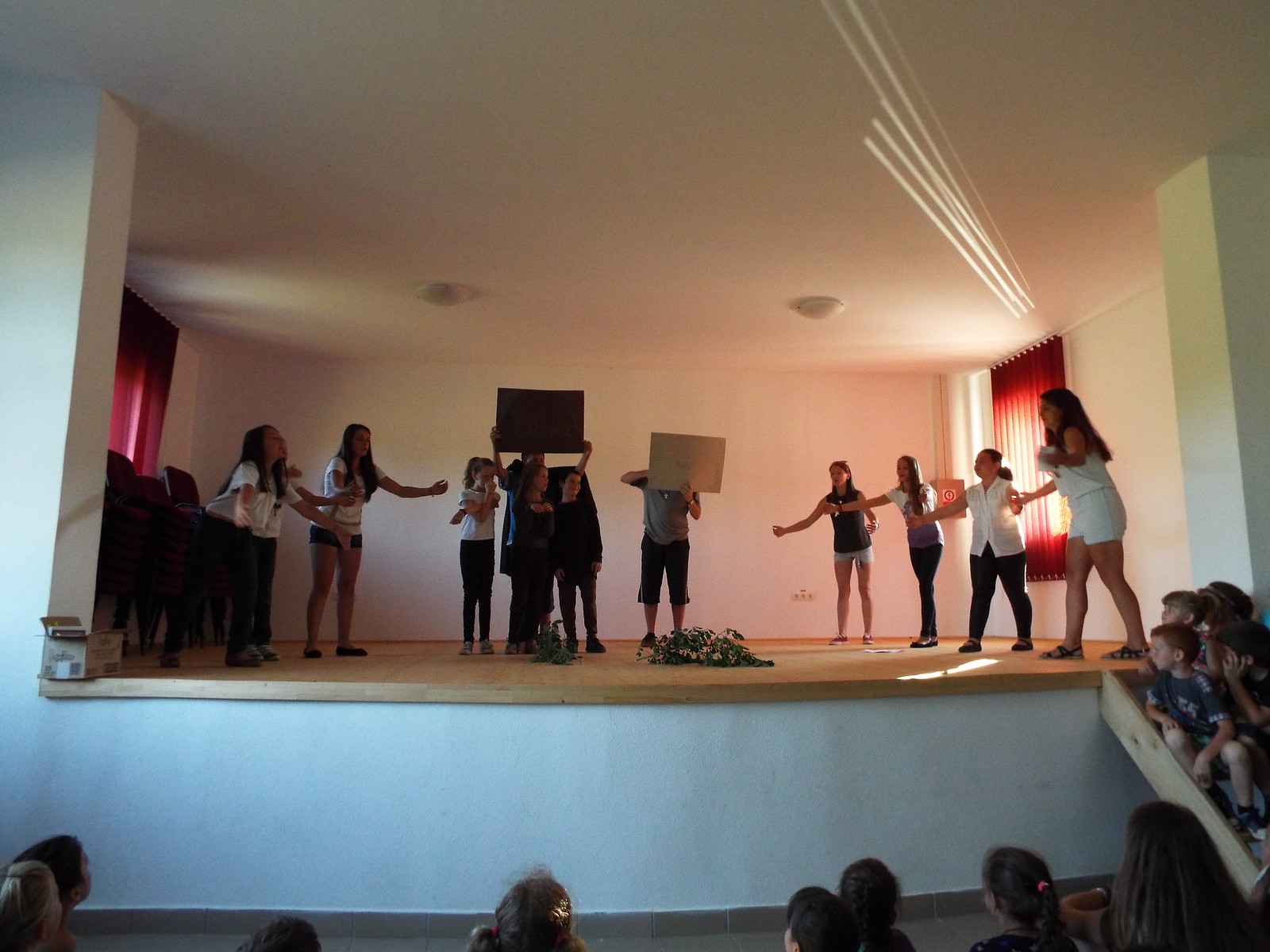This landscape-oriented color photograph captures a dynamic scene of young performers on a stage amidst a theatrical or musical rehearsal. The stage, featuring a honey oak finish floor and white rounded front wall, hosts approximately 12 individuals of varying ages, predominantly teenagers, arranged in small groups. Central to the scene are performers holding up blank cardboard signs, hinting at a possible guessing game or scripted routine. Some performers have their hands raised towards the sign-bearers, suggesting a coordinated group activity. Sunlight, rather than stage lighting, bathes the venue, creating natural illumination. The background is adorned with branches and leaves, adding a touch of nature to the performance setting. The audience consists of young children, estimated to be seven or eight years old, whose heads are visible from the back at the bottom of the photograph. Additionally, several children are seated on wooden stairs to the right side of the stage, all intently watching the ongoing rehearsal.